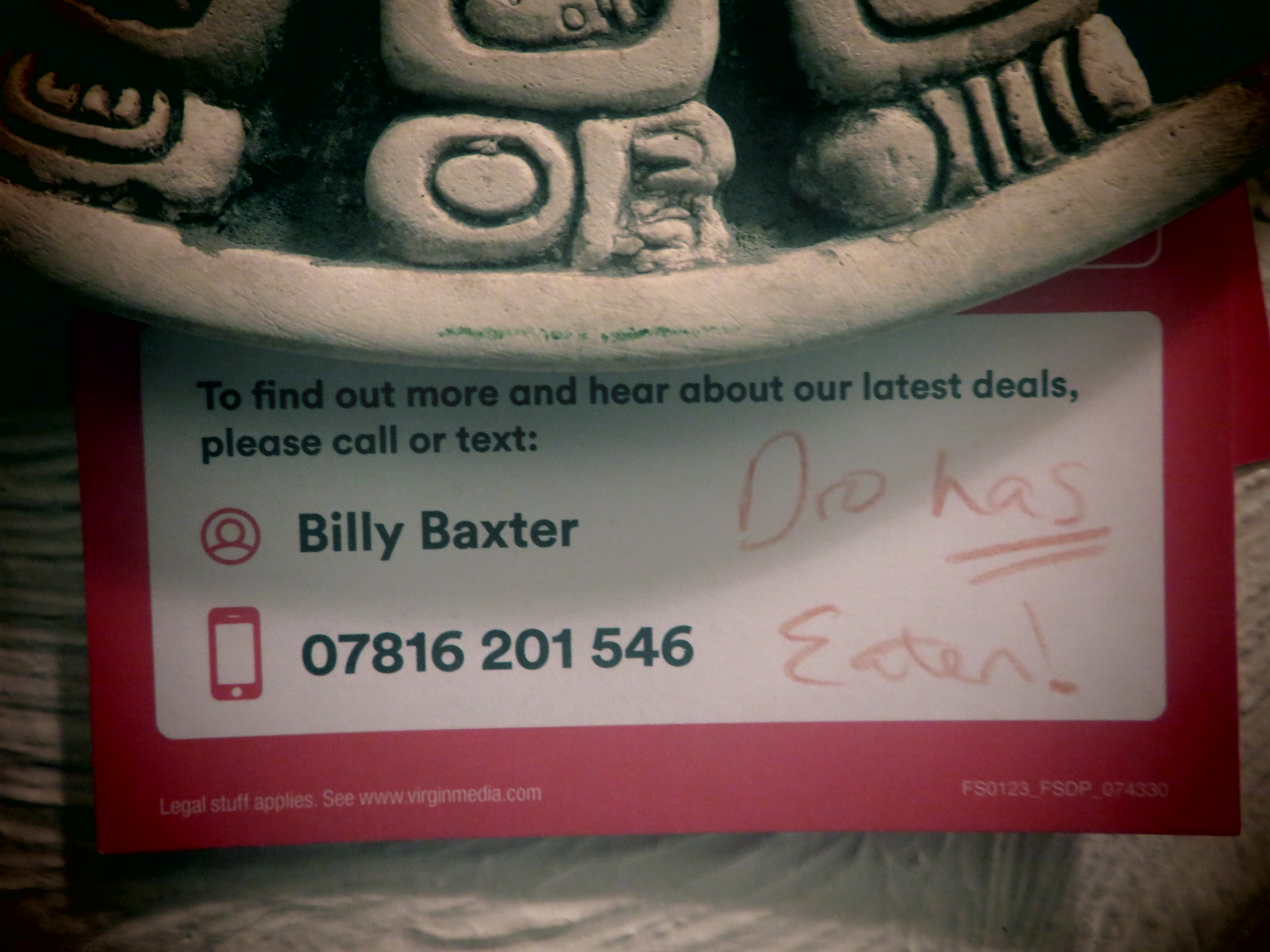The image features an up-close photograph of a stonework statue, possibly a lid, adorned with various designs and circular engravings. Positioned below the statue is a red business card primarily dominated by a white rectangular bubble in the center. The card reads, "To find out more and hear about our latest deals, please call or text." In black text, it mentions "Billy Baxter" beside a red icon of a person. Below this, another red icon depicts a mobile phone, positioned next to the black text "07816-201546". On the right side of the card, against a darker background, there is handwritten text in red, possibly resembling crayon, stating "DRO has eaten" with an exclamation mark emphasizing "eaten". The stonework background extends around the card, adding texture and depth to the image.